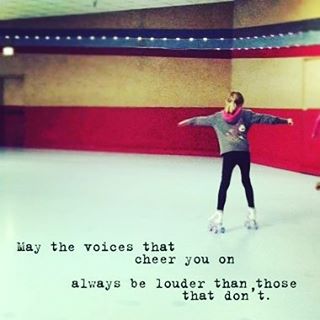The photograph captures a young girl standing in the middle of a roller rink, taken from behind. She appears to be learning how to skate, with her arms stretched straight out to her sides for balance. She is dressed in a gray sweatshirt with an indistinct picture on the back and a pink hood, paired with black pants. Her blonde hair is tied up in a ponytail. She wears white roller skates with gray wheels. The roller rink has a smooth, white floor, giving it an icy appearance, and the walls are distinctly color-blocked: the lower part is red up to about four or five feet, followed by a tan section, and topped with light blue and red stripes. At the bottom of the image, a motivational message reads, "May the voices that cheer you on always be louder than those that don't."